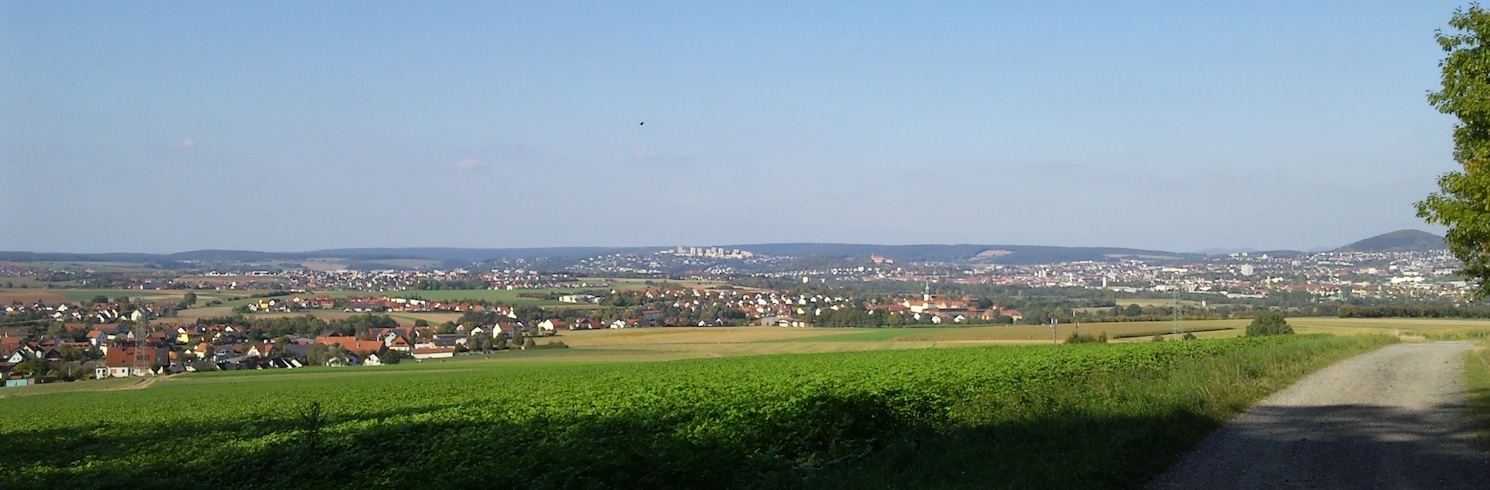The image captures a picturesque outdoor setting dominated by a brilliant, clear blue sky, free from clouds but with a slight haze. The foreground showcases a lush grassy field, vibrant and green, indicative of spring, with prominent shadows cast by tree branches on the left. To the right, a walking pathway—possibly gravel or concrete—partly disappears into these shadows. Tree branches with green leaves peek from the right edge of the frame. Beyond the field lies a sprawling view of distant houses and neighborhoods, interspersed with further patches of green. The background features mild hills transitioning into a single prominent mountain on the right, all blending subtly under the atmospheric pressure effect as they recede toward the horizon. This serene scene is warmly lit, suggesting a time later in the day.